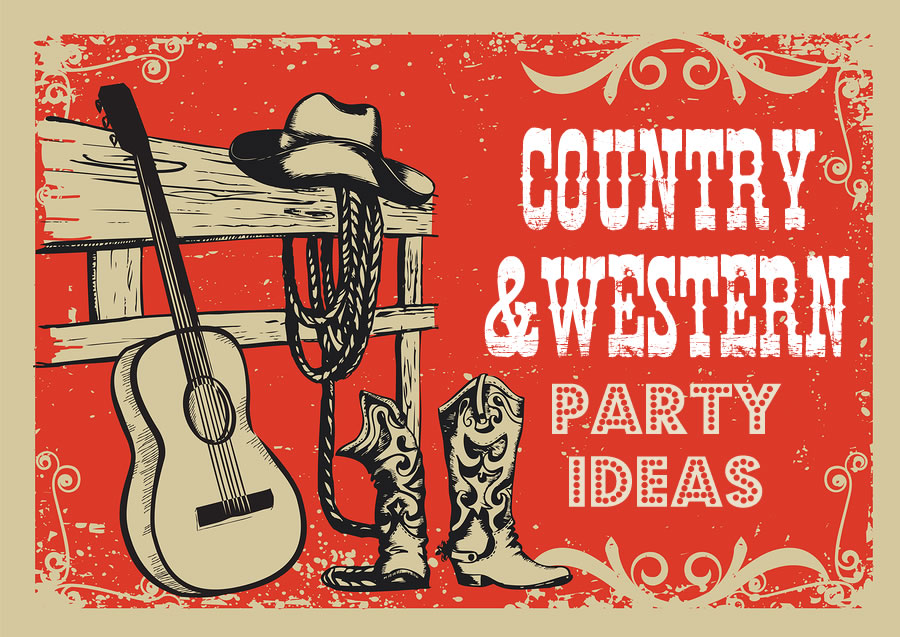The image is a rectangular print piece featuring a simple multi-color design with a beige (or light brown) border. The background is speckled red with gray intermixed. In the top right corner, the text "Country and Western" is written in white western-style font, and just below it, "Party Ideas" is displayed in a lit-up, neon sign font with red circular dots inside each letter. 

On the left side, there is a wooden fence adorned with iconic country-western elements. A cowboy hat rests on the top rail, with a lasso looped around it. A pair of empty cowboy boots sit below the rail, and an acoustic guitar is leaning against the side of the fence. The overall aesthetic is enhanced with ornate decorative swirls in the corners, capturing the essence of a stereotypical country-western scene. The image is vivid and clear, with the setting brightened by natural light.